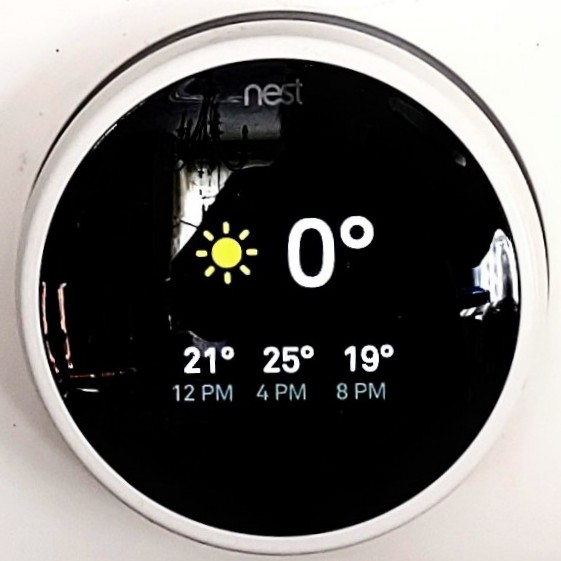This image features a Nest thermostat, prominently displayed against an off-white surface. The thermostat is round, encased in a thin, white metallic rim that contrasts elegantly with the surrounding wall. At its center is a glossy, black circular display, on which the word "Nest" appears at the top in small, precise letters. 

Beneath the brand name, there is an icon of the sun, represented by a circle with radiating lines. Below the icon, the current temperature is indicated as "0°". The display also shows a schedule: 21 degrees at 12 PM, 25 degrees at 4 PM, and 19 degrees at 8 PM. Reflections of light from a nearby window can be seen in the black display, adding a dynamic touch to the sleek design.